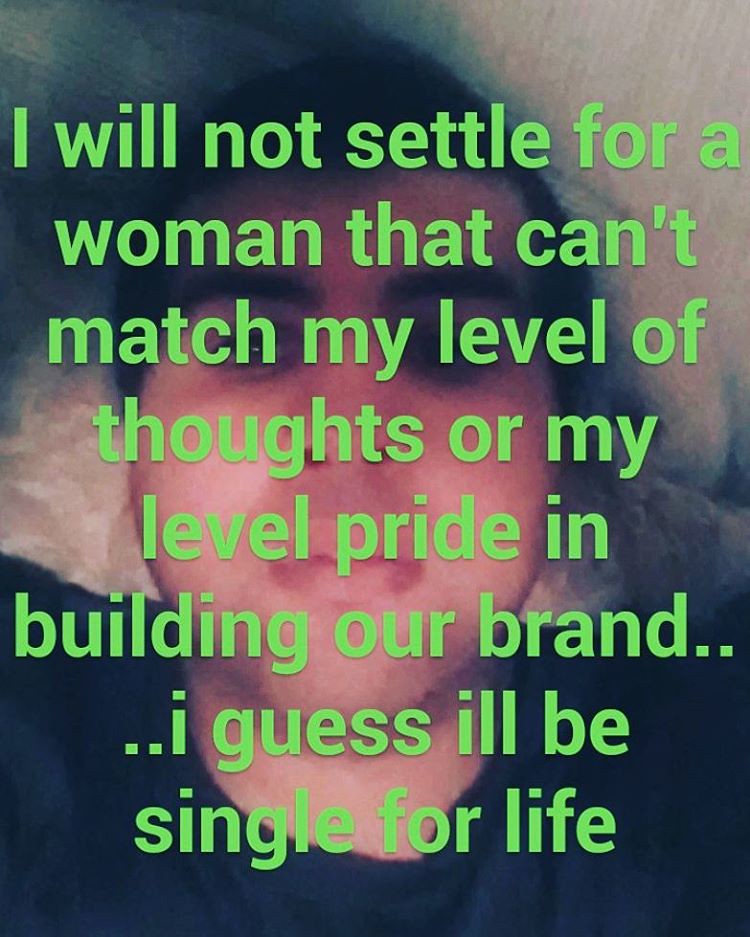The image features a young man, likely in his late teens, taking a close-up selfie while lying under a blanket or sheet. His dark hair and eyebrows frame his face, and he's wearing a blue shirt with a rounded collar. The background of the photo is slightly blurred. Overlaid on the image is a message in light green font that reads, "I will not settle for a woman that can't match my level of thoughts or my level of pride in building our brand. I guess I'll be single for life." The text is notable for its lack of punctuation and inconsistent capitalization, characteristics typical of social media posts. The message indicates the man's feelings of frustration and rejection related to his difficulty finding a suitable partner.